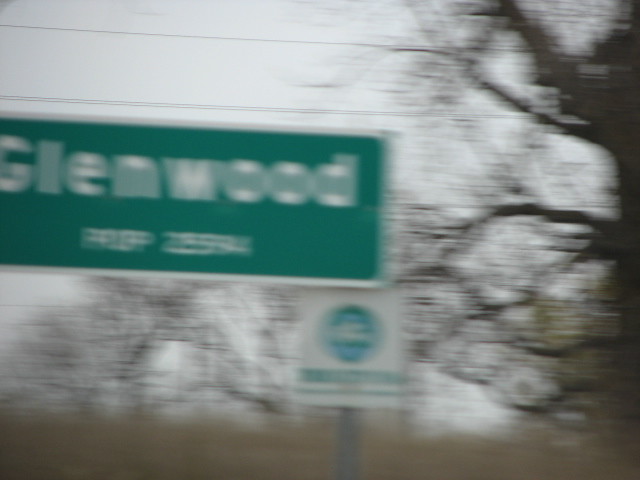This blurry, out-of-focus photograph appears to have been taken outdoors from a moving vehicle on a gray, overcast day. Dominating the image is a green rectangular road sign with white text that reads "Glenwood." Below this main sign is another, smaller white sign featuring some green text and a blue symbol, though its details are illegible due to the motion blur. Positioned on a silver post, the signs stand to the left-middle of the frame. In the background, a bare tree with broad branches is visible on the right side, alongside some other indistinct trees and long brown grass at the bottom of the frame. Overhead, power lines stretch horizontally across the gray sky, adding to the scene's sense of desolate motion.